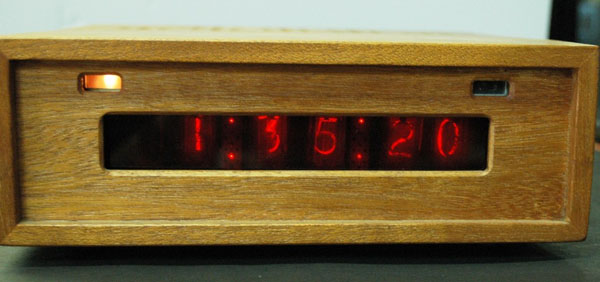The photograph features a close-up of a horizontally rectangular, brown plastic clock with a wood grain pattern. The clock is positioned on a gray or black table, taking up most of the horizontal frame, while the background at the top is a plain white wall. This clock is visually constructed to resemble a wooden box with horizontal wood grains. At its center is a black rectangular display that shows the time as "1:35:20" in bright red digital digits, reminiscent of an old digital watch. Above this main display, on the upper left side, there's a small rectangular area illuminated by an orange light, while a similar rectangular section on the upper right remains unlit. The natural lighting in the indoor setting accentuates the clock's detailed texture and colors.